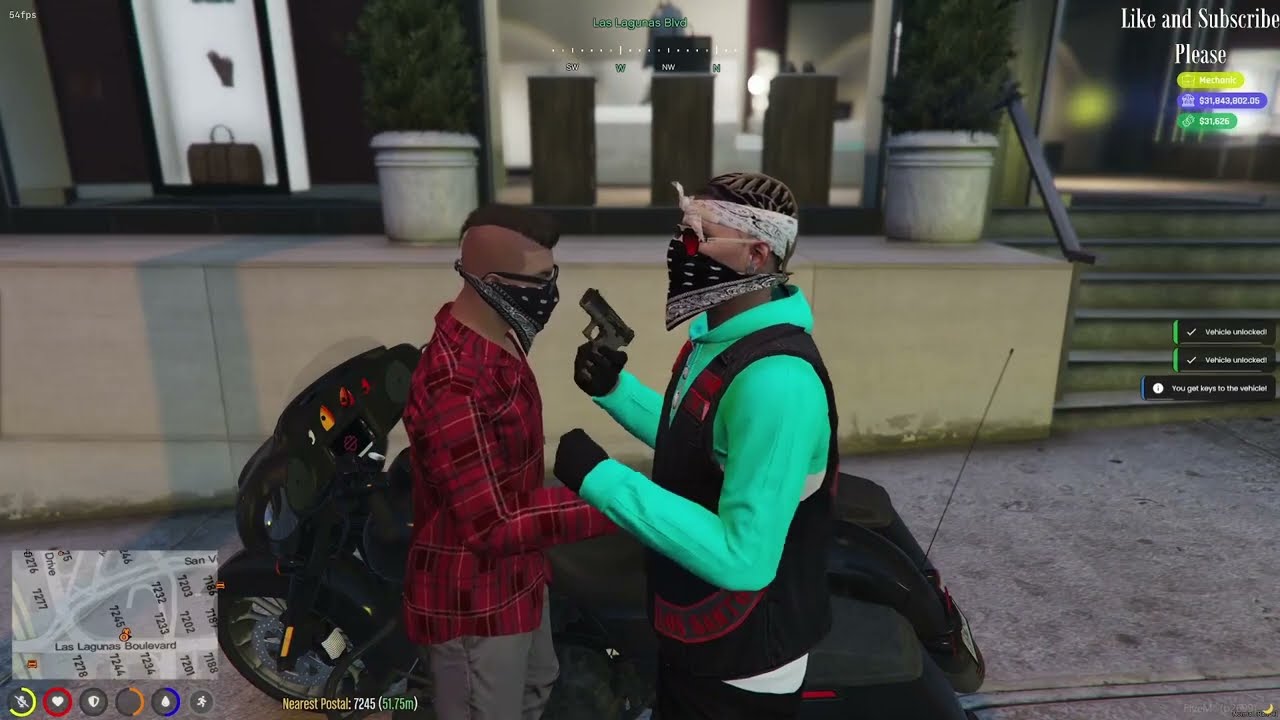This color photograph looks like a still shot from a video game, capturing two men in an intense face-off. Underneath a gray sky, they stand on a gray pavement, with a black motorcycle parked nearby. The man on the left, who appears to be Black with a black mohawk, wears a red plaid flannel shirt and gray pants. He has sunglasses and a black bandana covering his nose and mouth. He also carries a large black backpack. 

Facing him is another man with brown skin, wearing a neon blue hoodie under a black leather motorcycle vest with red patches. He has tightly woven braids, a white bandana tied around his forehead with the tie in front, and a black bandana over his nose and mouth. He completes his outfit with sunglasses featuring red lenses and black gloves. In his right hand, he holds a gun pointed towards the man on the left. 

Directly behind them is a black motorcycle with saddlebags, set against a gray stone wall with planters holding green trees, reminiscent of storefronts lining the background. A stairway leads to the upper right corner. The lower left corner of the image displays a mini-map typical of video games, with health stats beneath it. In the upper right, white text reads, "Like and subscribe, please."